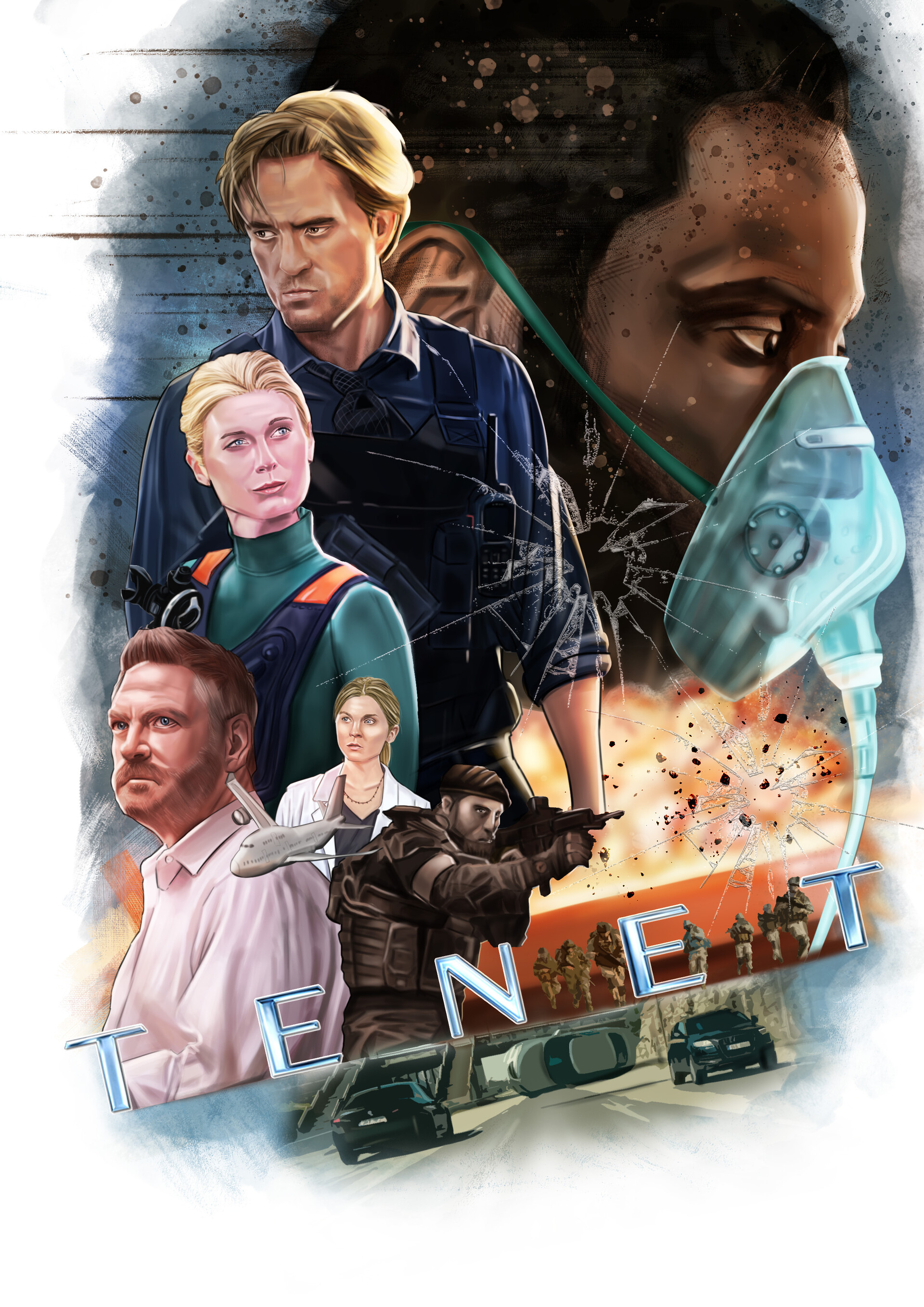This animated mural illustrates a dynamic scene from the movie "Tenet." At the bottom of the image, the title "TENET" is prominently displayed in a mix of white and blue text. Just below, a chaotic freeway scene unfolds with two black cars navigating in opposite directions while a white car flips on its side amidst the turmoil. The scene includes a tunnel in the background, intensifying the sense of action.

Above the freeway, the animation features six distinct characters. On the left, a black man is depicted wearing a blue hospital mask with a green tube extending down to the right side of the image. Next to him, a man in a white button-down shirt stands, followed by a woman in a green shirt paired with blue and orange overalls. A man in a blue button-down shirt is situated to the right, with his sleeve rolled up and blond hair visible. Another woman, donning a white jacket, is positioned further right. Above them all, a military individual with a drawn gun is visible, adding to the intensity of the scene. In the background, an explosion couples with the presence of other military personnel to amplify the chaotic and action-packed atmosphere of the image.